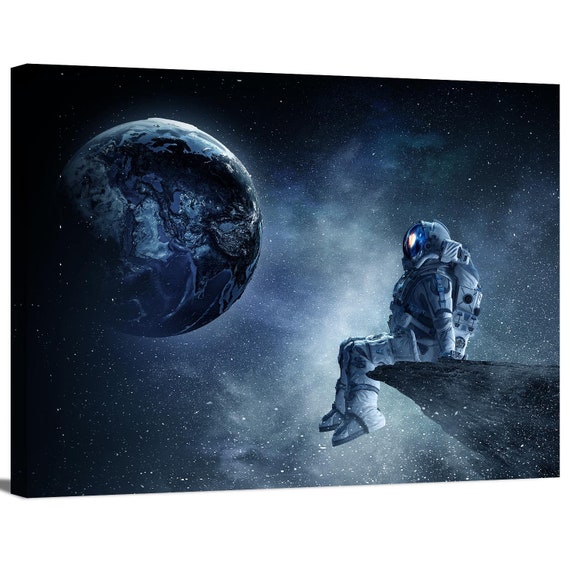An artistic rendering depicts an astronaut in a typical white spacesuit, complete with a helmet, life support pack, and white boots, sitting precariously on the edge of a sharply receding cliff or peak. The scene is set against the vast, dark expanse of outer space, characterized by midnight blue hues and Milky Way-like shading filled with stars and gaseous clouds. The astronaut gazes up intently at the distant, dimly lit planet Earth, which occupies the left half of the image. Earth is discernibly depicted with Africa, the Middle East, India, and Europe faintly visible despite the overall darkness. The composition exudes a dreamy, almost surreal quality, as if the astronaut is either trapped in space or simply taking a contemplative moment to look back at their home planet from the endless void.